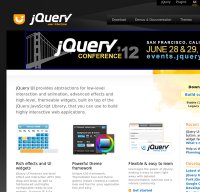This cropped image showcases the top left quarter of a web page dedicated to the jQuery Conference 2012, held on June 28-29 in San Francisco, California. The prominent area features a top banner, predominantly black, which houses the navigation menu. This banner contrasts sharply with the main page, which is primarily white with touches of an orange background adding a bit of vibrancy. The banner also includes a stylized silhouette of the iconic Golden Gate Bridge in white. The text on the page, though small and somewhat pixelated, delves into discussions on jQuery, exploring new features and developments related to web design and data tables. The page is rich in content, although this snippet cuts off midway through two sections, indicating that there is much more detailed information below.